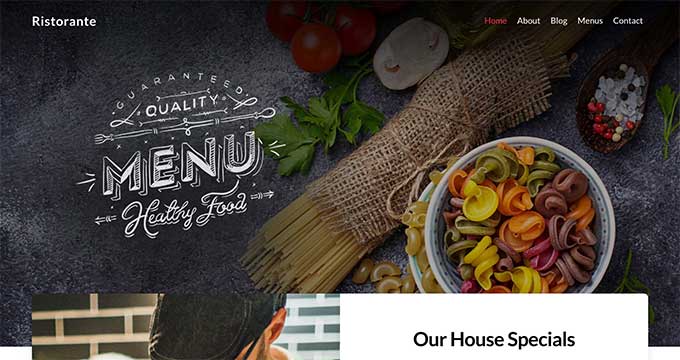In the top left corner of the image, the word "RISTORANTE" is prominently displayed. The background primarily consists of dark gray or black hues, providing a sleek and elegant backdrop. An emblem or sign in the upper section reads "Guaranteed Quality," emphasizing the restaurant's commitment to excellence. The word "MENU" appears in bold 3D letters, followed by the phrase "Healthy Food" beneath it.

To the right, a bundle of green herbs adds a fresh, vibrant touch. Adjacent to this, a straw container is filled with long, light brown pasta noodles, resembling spaghetti. Additionally, a bowl contains a variety of colorful, twirled, and curly pasta noodles in muted shades of orange, purple, yellow, and green.

Positioned underneath the bowl, the text "Our House Specials" is printed in black, guiding viewers' attention to the featured dishes. In the upper right corner, under the word "Home" in red, there are links labeled "About," "Blog," "Menus," and "Contact." Above the green herbs and near the phrase "Quality Menu," a cluster of two or three red tomatoes is depicted, enhancing the fresh and wholesome theme of the image.